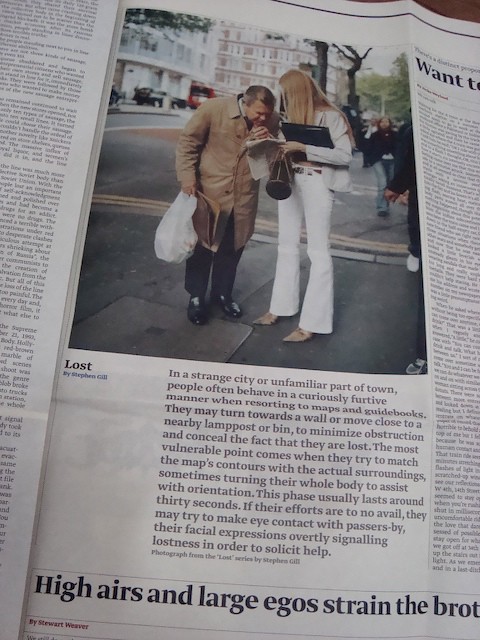This image captures a close-up photograph of a page from a likely newspaper or magazine, characterized by visible folds and several columns of fine print, with the central focus on a photograph and descriptive article. The prominent photo on the page features a man and a woman standing on a city street. The man, wearing a brown overcoat, black pants, and black shoes, is holding a briefcase and a white plastic bag in his right hand, while leaning forward to look at something the woman is presenting. The woman, dressed in a white jacket and white bell-bottom pants with pointed heels, holds a black portfolio and possibly a newspaper with her left arm. The street setting includes dark gray asphalt, bordered by a curb, with visible residential buildings, vehicles including a potential bus in the distance, and pedestrians.

Below the image, a caption titled "Lost" by Stephen Gill describes the typical behavior of people who are lost in unfamiliar environments, emphasizing furtiveness and attempts to orient themselves with maps or guidebooks. The caption notes how individuals might turn their whole body to match maps to their surroundings and may seek help from passers-by through eye contact and facial expressions signaling their disorientation. The photograph is credited to Stephen Gill as part of his "Lost" series. To the right of the main text is another article snippet beginning with the word "Want," while at the bottom, another headline partially reads "High Heels and Large Ego Strain the Brotherhood" by Stewart Weaver.